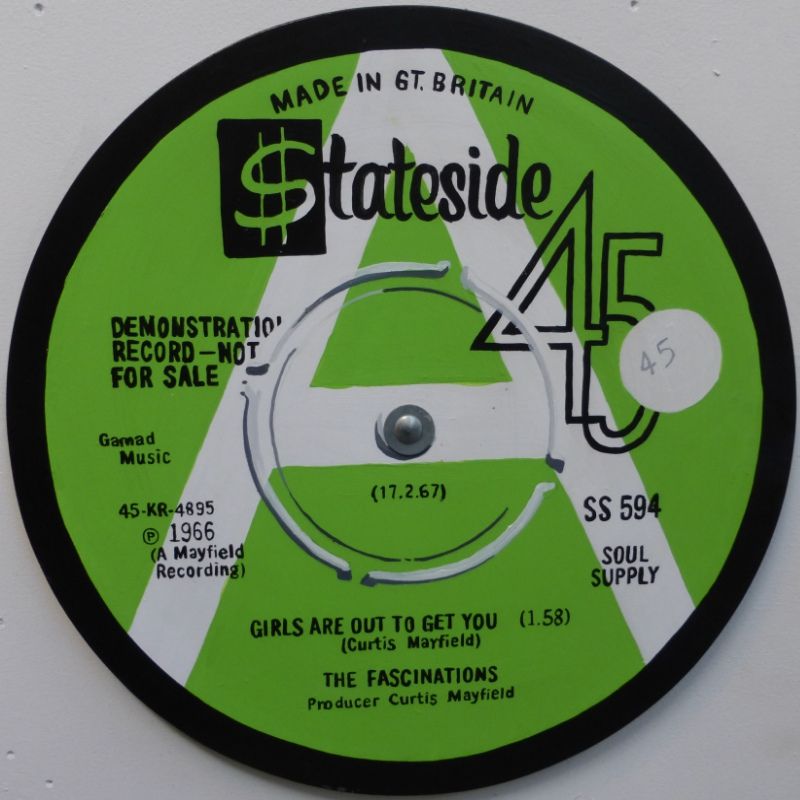The image displays a vinyl record with a light green label featuring a large white letter 'A' at its center. The text on the label is primarily in a brushy, handwritten-style font, though somewhat uneven. The label is branded "stateside" with the first 'S' represented by a dollar sign. The record, marked as a "demonstration record, not for sale," indicates it was "made in Great Britain," with 'Great Britain' abbreviated as "GT Britain." Additional text includes "Garwad music," "45KR4895P1966A," and a Mayfield recording date "17.2.67." The listed tracks are "Girls Are Out To Get You" by Curtis Mayfield and The Fascinations, stating Curtis Mayfield as producer, alongside catalog details such as "45SS594" and "soul supply."